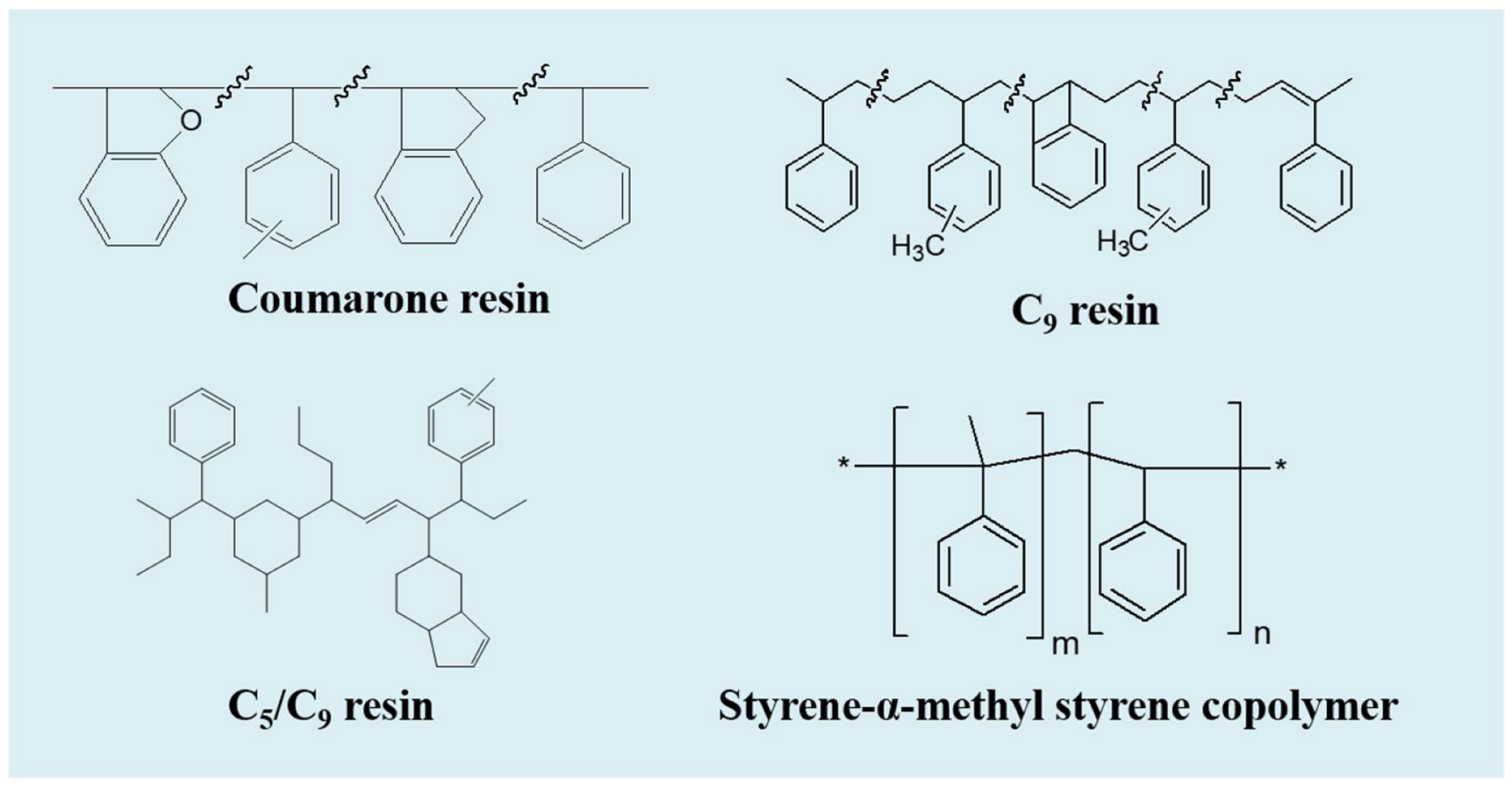The image portrays a light blue background with meticulously drawn molecular structures of four distinct organic compounds, each labeled and detailed in different segments of the poster. 

In the top left corner, labeled “coumarin resin,” multiple interconnected hexagonal rings form complex patterns. This section additionally includes the notation “C9 resin” alongside detailed molecular lines, such as the H3C group depicting three hydrogen atoms bound to a carbon atom.

Further down the left side, an area marked “C5-C9 resin” features five hexagonal rings arranged in a specific pattern where the rings alternate sides. 

On the bottom right, the label “styrene alpha-methyl styrene copolymer” presents another intricate molecular structure, displaying two rings within brackets and linked with various linear connections. Each molecular illustration employs black lines against the blue backdrop, providing a scientific representation of these compounds as they might appear in a laboratory setting.

Across the entire image, these molecular diagrams, composed of hexagonal forms and linear connectors, collectively offer a detailed visual representation of the chemical compounds: coumarin resin, C9 resin, C5-C9 resin, and styrene alpha-methyl styrene copolymer.